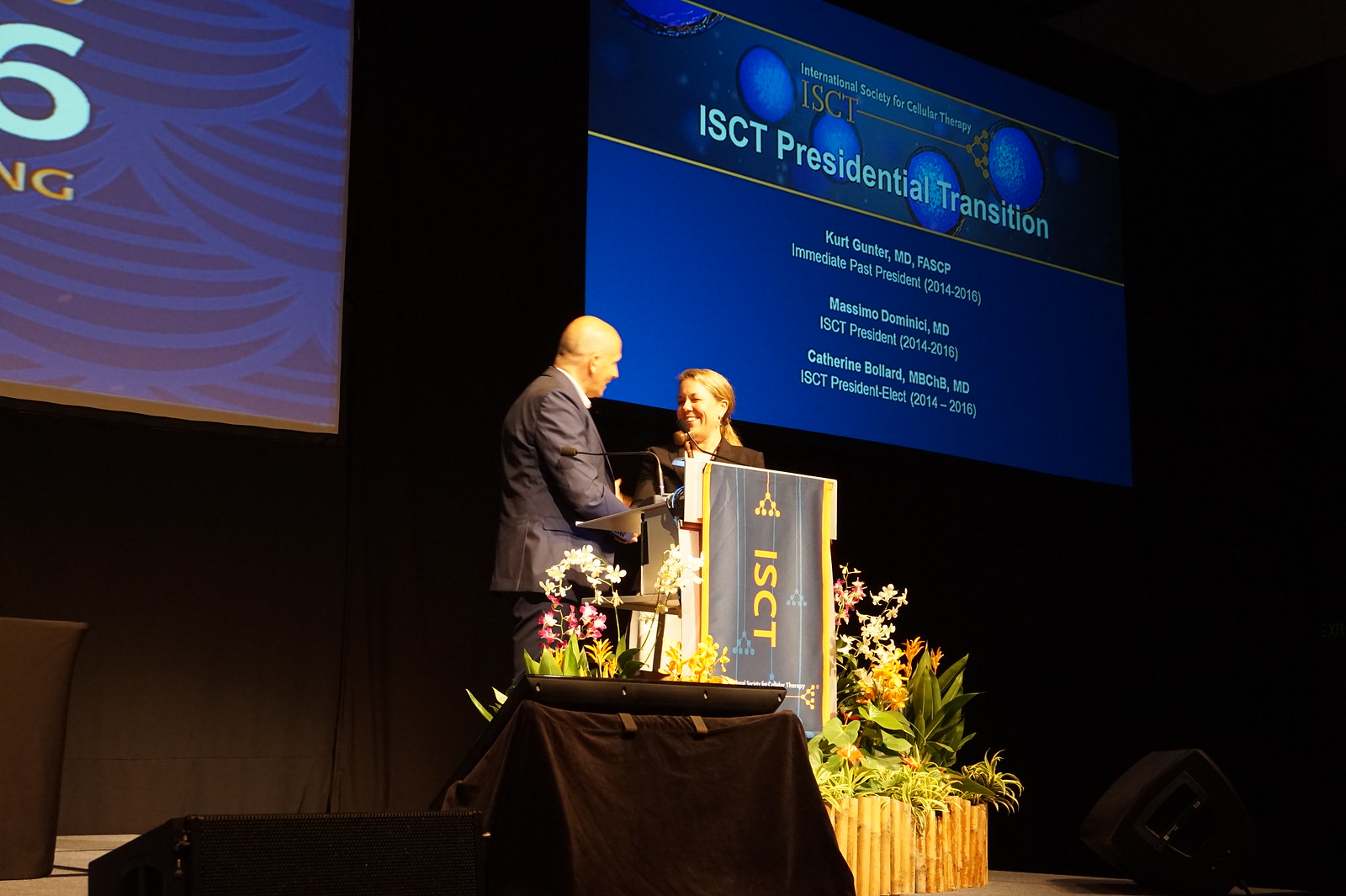In the image, two individuals are prominently standing at a podium centered on a stage, engaged in what appears to be an award presentation or a ceremonial speech. The man on the left, who is wearing a blue suit with a white collar and is bald, is smiling broadly at the woman on the right. She has blonde hair styled in a ponytail and is also smiling warmly. Both are positioned directly in the center of the photo, shaking hands. The podium they stand behind features a sign that reads "ISCT," with an array of decorative flowers around its base.

The setting is indoors, with the photograph taken at a slight diagonal angle, revealing a stage background that includes two large screens. The screen at the upper right clearly displays the words "ISCT Presidential Transition" along with the names Kurt Gunther, Massimo Damanisi, and Catherine Ballard, against a predominantly blue backdrop. The other screen, located at the upper left, is also predominantly blue but is partially cut off, making its contents indistinguishable. The overall color scheme in the image includes shades of brown, gray, white, yellow, green, tan, blue, and orange. The context, indicated by the screens and formal attire, suggests this is a professional conference or medical seminar, spotlighting an important transition within the ISCT organization.